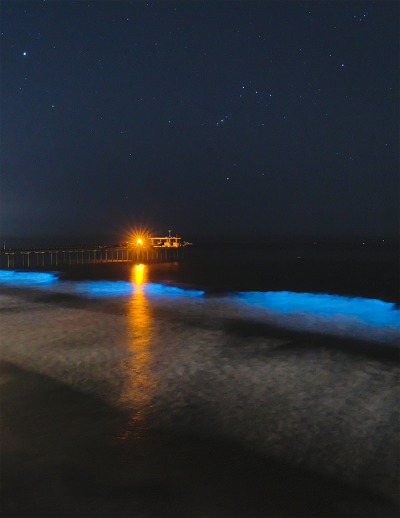In this nighttime seascape, the ocean meets the seashore diagonally from the center-left to the lower right of the frame. The dark gray night sky is punctuated by a few white stars, casting a serene, almost haunting atmosphere. To the left, a brown pier extends from the center-left towards the center, ending in a building emitting a glowing, bright yellow light with an orange halo. This light casts a striking reflection across the water and the sandy shore in a straight orange line. The shoreline reveals a mix of tan sand with patches of dark brown shading. Where the waves meet the beach, the water glows a captivating bioluminescent blue, contrasting sharply with the nearly black ocean beyond.